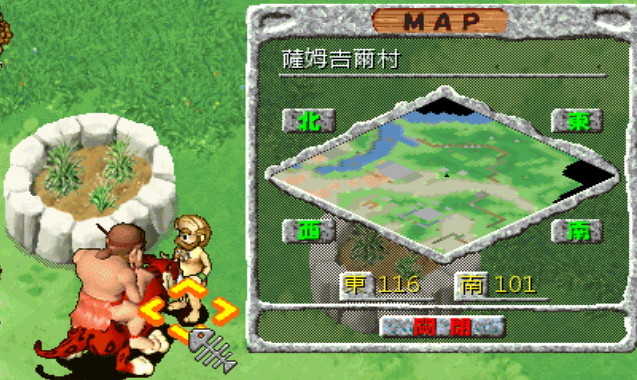This screenshot from a vintage video game features a richly detailed scene. The right side of the horizontally long image is dominated by a large, rectangular gray stone structure that spans from nearly the top to the bottom of the screen. At the top center, there's a wooden label that reads "MAP" in black English letters. Beneath the label, the map area displays a diamond-shaped arrangement reminiscent of games like Starcraft or Warcraft. This map has intricate details, including water, green grass, and buildings, surrounded by gray stone rectangles marked with green Chinese symbols.

Below the map, to the left, two smaller gray stone squares display the numbers 116 and 101 in Chinese characters. Adjacent to this setup, there is another narrow rectangular stone with additional Chinese symbols.

To the left of this central map area, the background transitions to green grass scattered with various objects and characters. In the bottom left corner, two shirtless, cartoonish caveman characters are depicted; one character, wearing a red loincloth, is riding a brown and black spotted animal with white paws, possibly a leopard. This character is shown from the back, while the other caveman, facing forward, appears to be engaging in some sort of battle.

Notably, the foreground features a well-like stone circle containing dark brown dirt and green plants, situated at the bottom of the map area. Additionally, nearby on the ground are a fish skeleton and an orange circle, possibly a video game selector.

Overall, this image captures the essence of a classic video game scene with its detailed map, engaging characters, and a blend of text in both English and Chinese.